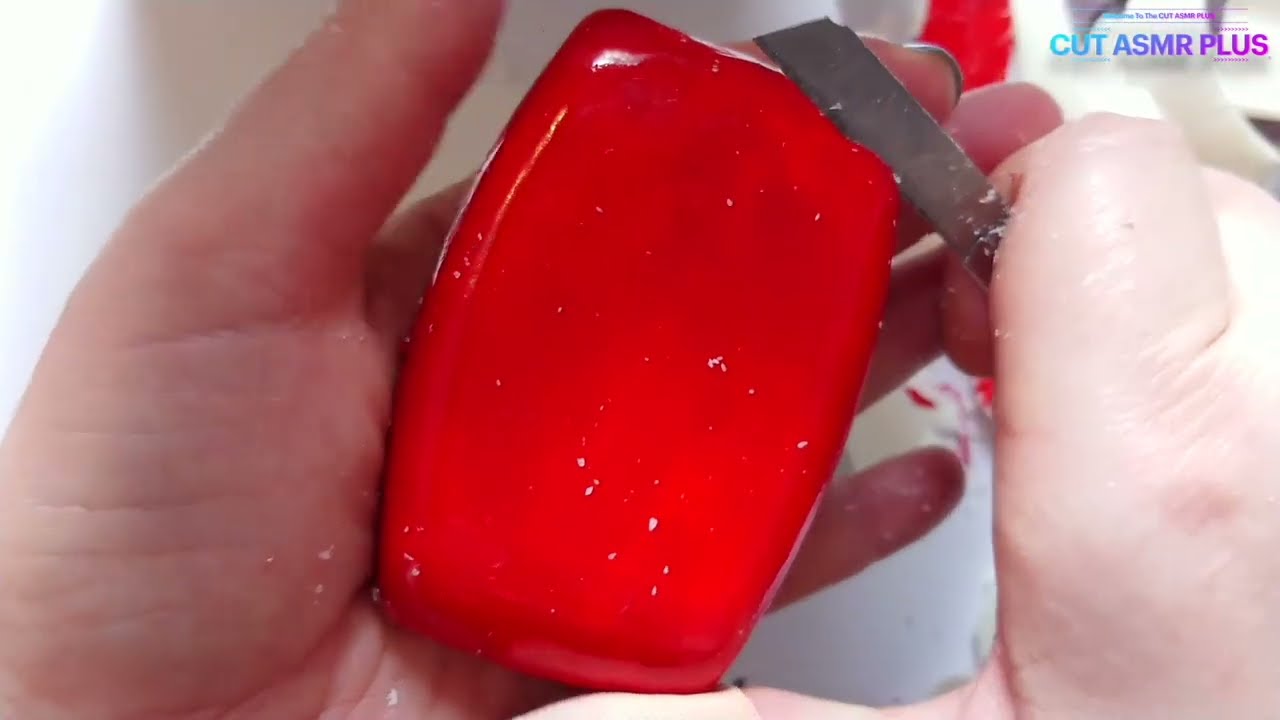This is a highly detailed, full-color screenshot captured from an ASMR video featuring the logo "Cut ASMR Plus" in the upper right corner, with text that transitions from teal to purple and pink. The horizontally rectangular image showcases a pair of Caucasian hands, one of which holds a bright red, translucent rectangular object that appears to be a bar of glycerin soap. The hand holding the soap is oriented with the palm side towards the viewer and is covered in white flecks, indicating that the soap has been partially shaved or carved. The other hand, with at least one dirty fingernail, wields a small gray razor blade poised to slice into the soap. The soap, with black metal or strap-like elements visible on its surface, is the focus of the scene, invoking the sensory experience typical of ASMR content through the sound of its slicing and scraping.